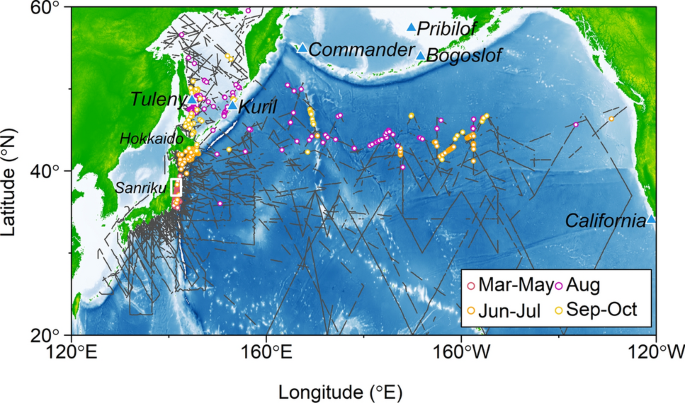This close-up scientific drawing is a detailed geolocation map of the Pacific Ocean spanning from the coasts of Asia and North America. The x-axis is labeled longitude and ranges from 120° East to 160° East, and from 160° West to 120° West. The y-axis is labeled latitude, covering 20° North to 60° North. The map features several distinct geographic locations marked by names such as Hokkaido, Sanriku, Tuleni, Coreal, Commander, Pribilov, Bogoslav, and California.

In the central region of the map, primarily a light blue area representing the ocean, numerous colored dots indicate specific points of interest or data, particularly in yellow and pink hues. These dots are cross-referenced with a legend located in the bottom right corner, which explains that pink dots represent data from March to May, while yellow covers June to July, and orange dots indicate September to October.

The image also displays potential maritime trade routes or travel paths with dots and lines spanning from Japan to California, suggesting the movement of ships across the ocean. The top of the map includes labels with blue triangles such as Commander, Pribilov, and Bogoslav, emphasizing specific locations, while the bottom right corner clearly marks California along the West Coast of the United States. The map encompasses the eastern tip of Asia on the left and the western coast of North America on the right, integrating critical points of interaction across the Pacific.